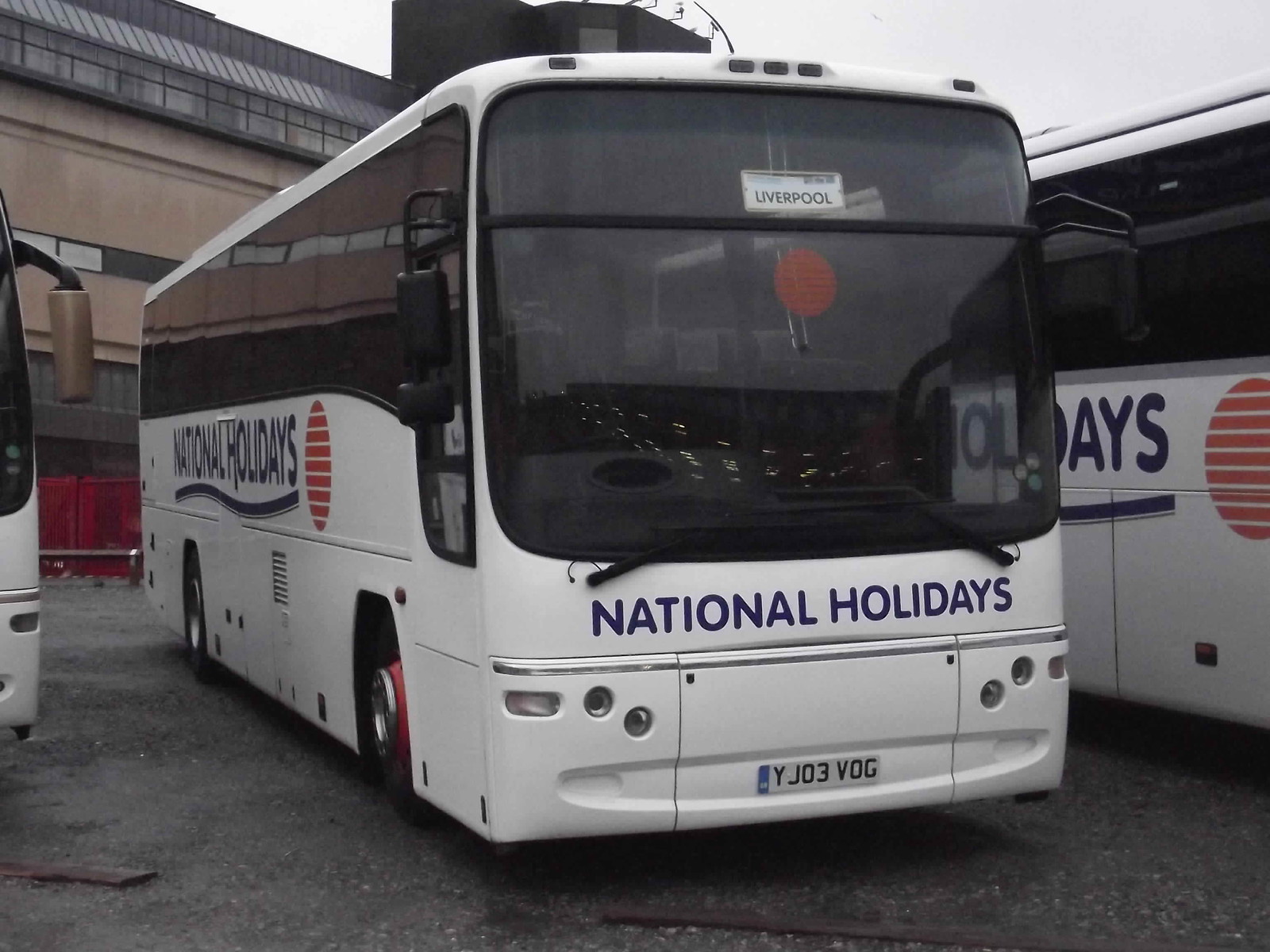This outdoor photograph features three National Holidays tour buses parked side by side in a lot, centered around the front and partial left side of the middle bus. All three buses are predominantly white, adorned with the "National Holidays" branding in dark blue capital letters on both the front and sides. The middle bus has a paper sign in its windshield reading "Liverpool." The buses have a flat front design with chrome accents and are nearly identical, including the distinctive red circle logo composed of horizontal stripes on their sides.

The background reveals an industrial-looking building with a tan facade and gray roof, featuring windows and possible black railings or window frames. Despite some ambiguity about the building's purpose, it adds an urban context to the scene. The skies above are gray, contributing to the overall somber tone of the photograph. The clarity of the buses’ branding and the symmetry of their arrangement highlight the organized nature of this scene, likely captured at a bus depot or similar facility.